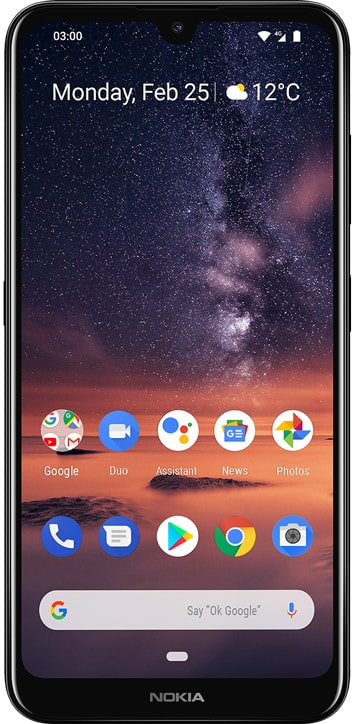This image showcases a Nokia Android smartphone from the front, highlighting its home screen. The Nokia branding is prominently displayed at the center bottom of the phone. The status bar at the top indicates the time as 03:00, with icons for wireless connection, cellular signal, and battery status on the right. Below the status bar, the date is shown as "Monday, February 25" in white text. 

The screen also features a weather widget displaying a partly cloudy condition with the temperature marked as 12°C, accompanied by an illustration of a cloud with the sun peeking behind it. The background image appears to be a dynamic sunset scene with a gradient blend of colors, possibly depicting a beach below, adding a tranquil aesthetic touch to the screen.

The app icons are arranged in a neat grid. The first row includes:
1. Google: An icon showing four colored dots.
2. Google Duo: A blue icon with a video camera symbol.
3. Google Assistant: An icon with multicolored circles.
4. Google News: An icon labeled "News."
5. Google Photos: An icon labeled "Photos."

The next row features:
1. Phone: Traditional phone handset icon.
2. Messaging: Text message icon.
3. Google: Classic Google "G" logo on a white background.
4. Google Chrome: Icon featuring the Chrome logo.
5. Camera: Camera icon.

Below these icons, there is a text search box with the Google logo and the prompt "Say 'OK Google'," suggesting voice search capability.

Overall, the phone's display is a blend of functional information and vivid imagery, providing a visually pleasing and efficient interface.